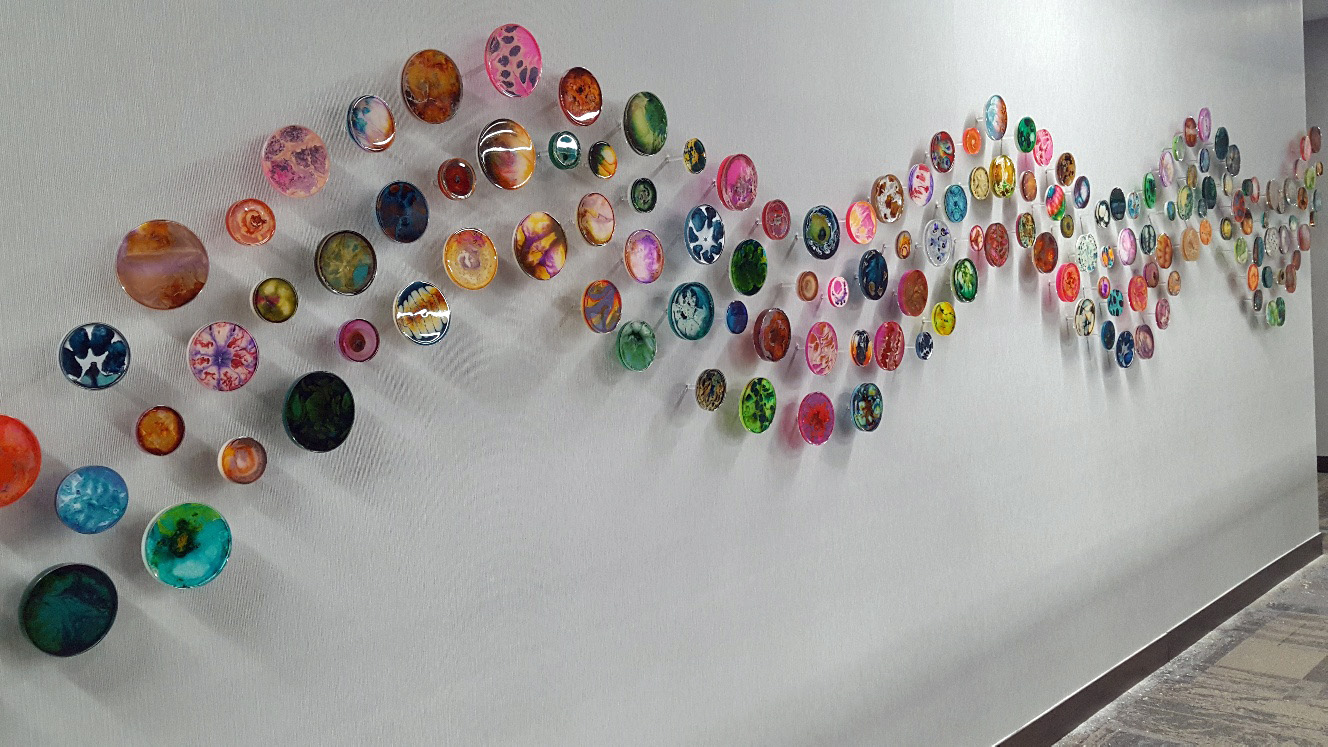The image depicts a modern art installation on a white wall, with the right side more brightly illuminated than the left. The wall features a wave pattern of round, crystal-like knobs in diverse colors and abstract designs—blue, orange, yellow, green, purple, and pink—resembling decorative furniture knobs or vibrant magnets. These knobs cascade in an undulating arrangement, varying between three and four rows high. At the base of the wall, there's a brown wood trim, and the visible floor is a laminate or linoleum with streaks of dark gray. The far right side of the image offers a glimpse of another room beyond the wall's end.